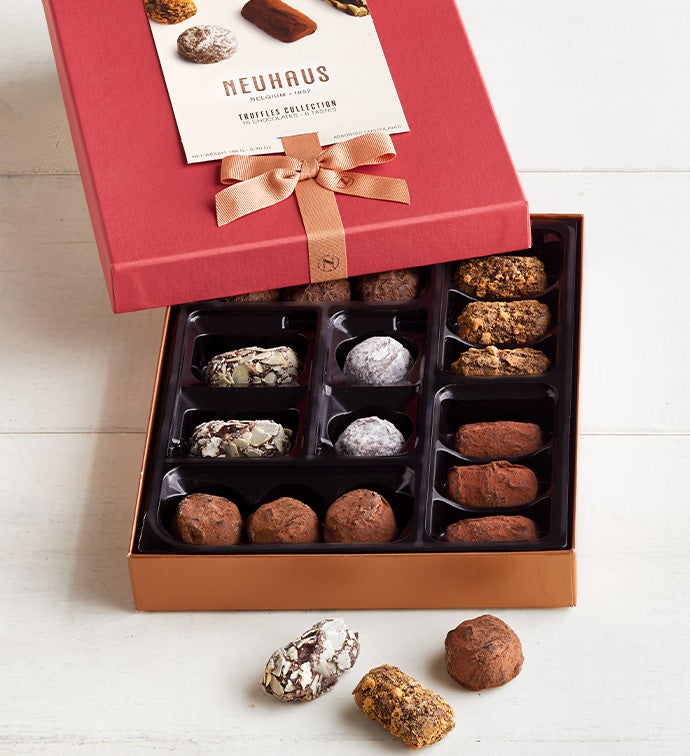A meticulously designed gift box showcases an exquisite assortment of Neuhaus chocolates. The square box features striking orange sides and a black plastic interior that securely nests each delectable truffle. The top of the box is a bold red, elegantly adorned with an orange ribbon and a sophisticated bow. Attached is a brochure labeled "Neuhaus Truffle Collection, Belgium, 1959," with some very fine, indecipherable writing at the bottom. The ribbon is further embellished with a logo—an 'N' encased in a circle—indicative of the Neuhaus brand.

Inside the box, each truffle is meticulously placed in its designated slot within the plastic mold. In front of the box, three truffles lie loose: one spherical truffle dusted with cocoa powder, and two cylindrical truffles—one seemingly encrusted with crunchy caramel bits, and the other coated in chocolate with white nut fragments. The truffle selection further includes variations such as chocolates rolled in confectioner's sugar and elongated versions of the cocoa-dusted round truffle, hinting at different enticing fillings. This luxurious collection invites chocolate aficionados to savor the rich heritage and craftsmanship of Neuhaus.